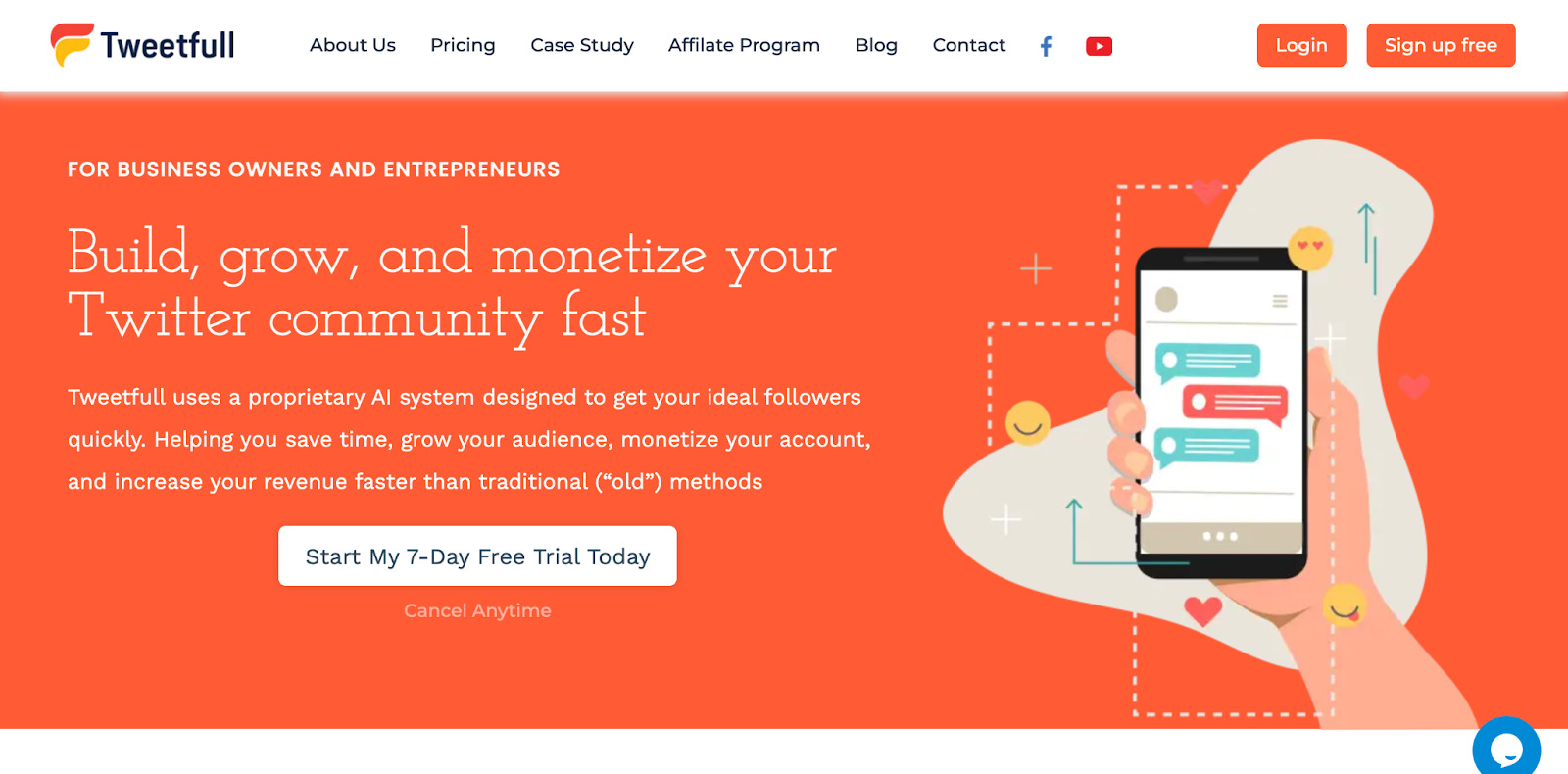In the upper left corner of the image, there is a curved orange line paired with a curved dark yellow line, next to which is the word "Tweetful." Below this header, there are several navigation options including "About Us," "Pricing," "Case Study," "Affiliate Program," "Blog," and "Contact." Additionally, a Facebook icon (represented by an 'F') can be seen here. 

To the right of these options is a red rectangle featuring an arrow icon. Adjacent to it are two orange rectangles, one labeled "Log In" and the other "Sign Up Free." 

On the right side of the image, an orange rectangle contains a picture of a hand holding a phone. The background behind the phone image includes a subtle gray pattern with running dots, giving it a dynamic feel.

The main promotional text on the left side reads: "For business owners and entrepreneurs. Build, grow, and monetize your Twitter community fast." It continues, "Tweetful uses a proprietary AI system designed to get your ideal followers quickly, helping you save time, grow your audience, monetize your account, and increase your revenue faster than traditional 'old methods'."

Beneath this text, there's a prominent white rectangle that invites users to "Start my 7 day free trial today," with a note underneath stating, "Cancel anytime."